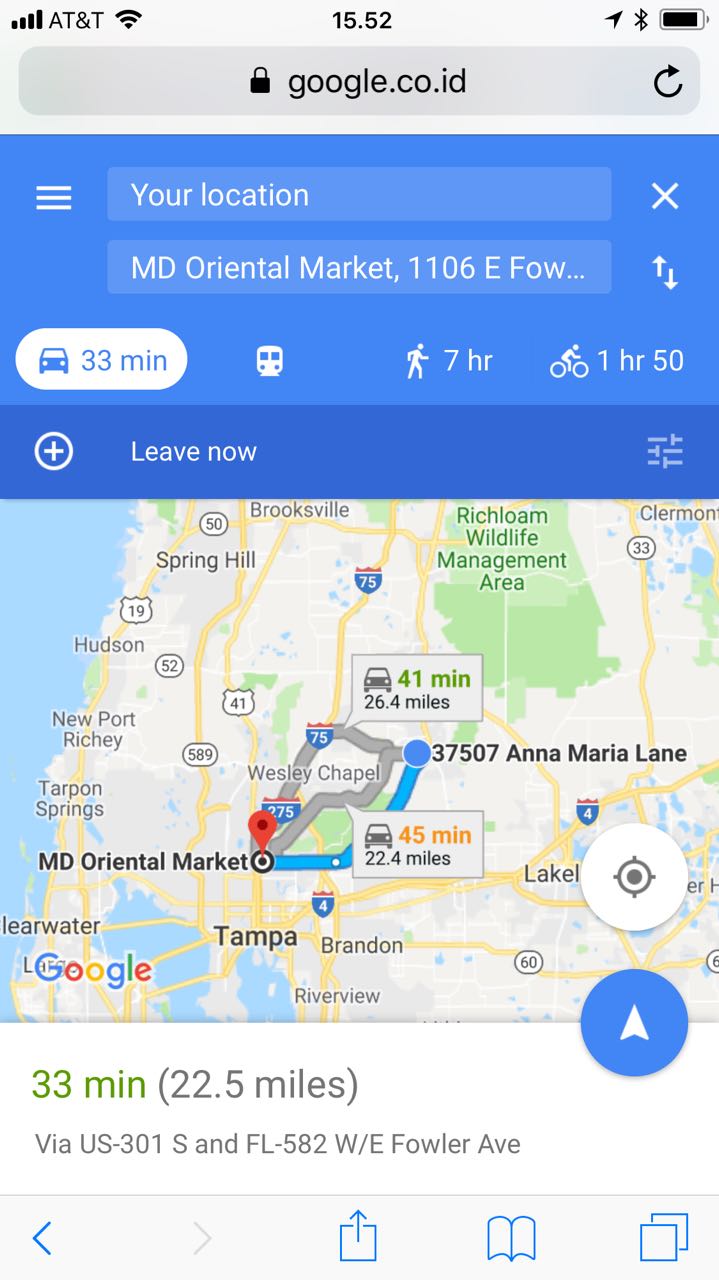This screenshot depicts a Google Maps interface on an AT&T smartphone, showing full signal strength with four bars and a Wi-Fi connection. The timestamp on the device is 15:52. The search was conducted on google.co.id, with the user's current location displayed at the top. The map centers around the MD Oriental Market at 1106 East Fowler Avenue, Tampa, Florida. Surrounding areas include Tampa's Annamarie Lane, Brandon, Riverview, Spring Hill, Hudson, Newport Richey, Tarpon Springs, and Brooksville, alongside a wildlife management area. The estimated travel time to the destination is 41 minutes, covering a distance of 26.4 miles.